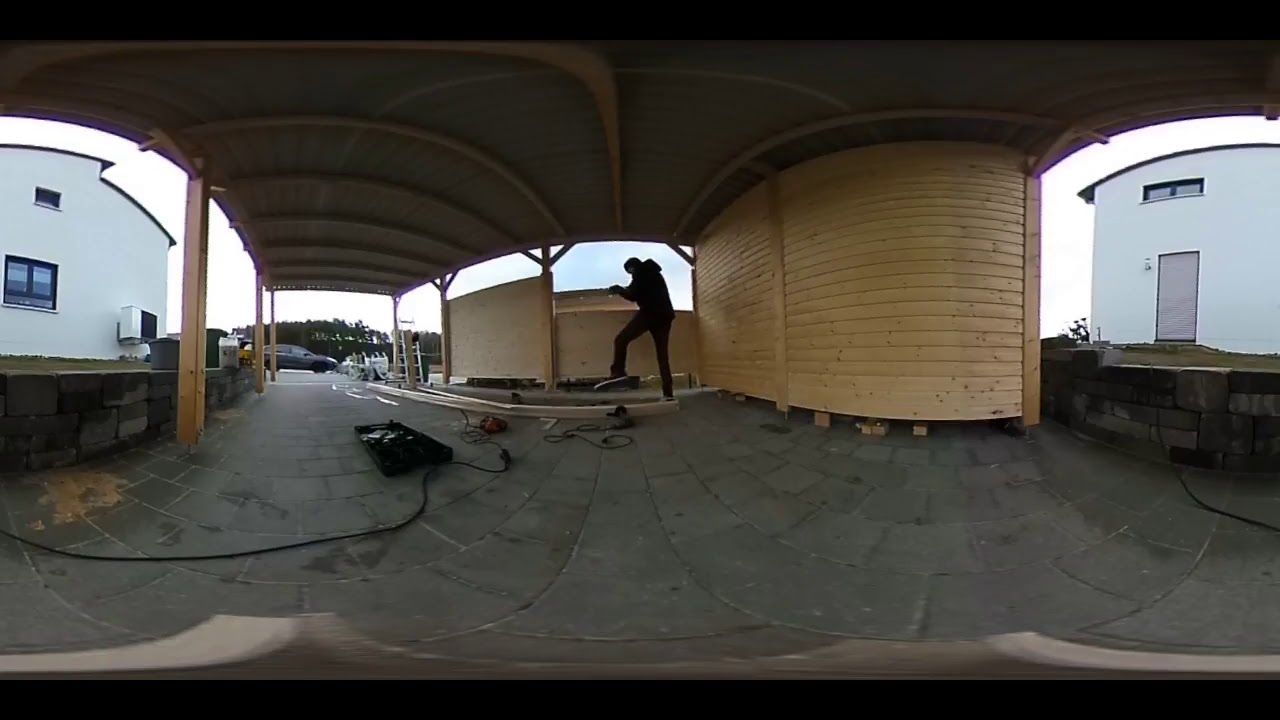The photograph is a color image capturing an outdoor, covered area with a roof supported by wooden pillars. The space appears to serve as a shed or a covered parking area, with an asphalt or stone-tiled floor and fully open sides. The image is horizontally aligned and bordered in black at the top and bottom. The scene looks somewhat warped and distorted due to its compression from a 360-degree format into a flat, two-dimensional view. 

On each side of this covered area, there are plain white buildings with black-trimmed windows and doors. The left building features a window at a lower level with an air conditioning unit attached. The right building has a small window above a gray door. Scattered across the floor are various cords and a black, rectangular object lying on the stone tiles.

A person dressed entirely in black stands towards the center. Although blurry and distant, they appear to be involved in some activity—possibly riding a skateboard and performing a stunt with one leg extended and arms raised, or working with the wooden wall nearby. More details, such as trees and a gray car parked in the distance, as well as an overcast sky, are visible beyond the covered area.